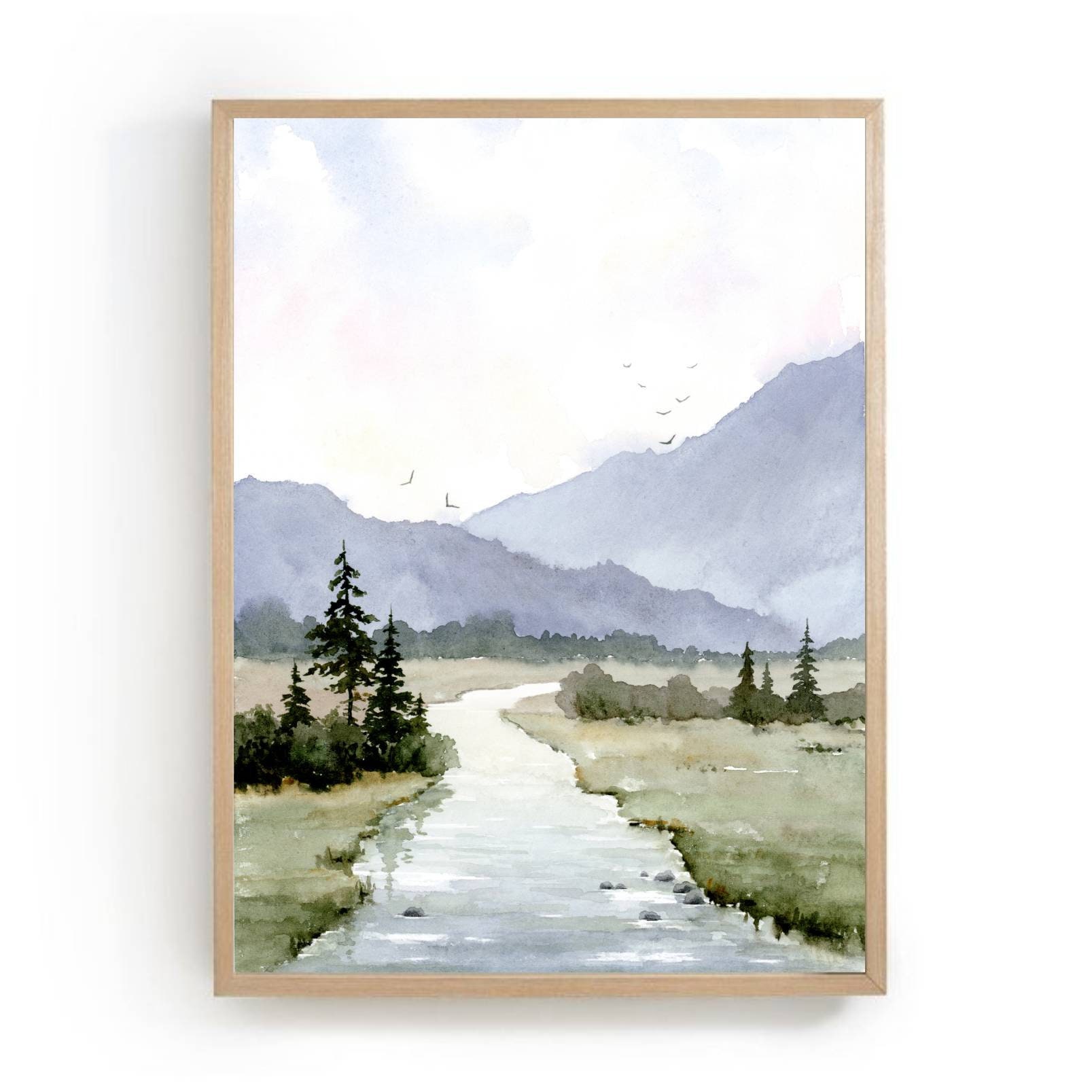This image is a detailed and serene watercolor painting housed in a tall, thin-bezeled, light wood frame. The painting beautifully captures a tranquil landscape featuring a softly winding stream that starts near the bottom left corner, proceeds upwards and to the right, and then curves back to the left before disappearing behind some greenery at the center. Green grasslands dominate the foreground, interspersed with clusters of dark, almost silhouetted trees on the left side and a mix of flat grassland and sparse trees on the right.

In the middle distance, the stream again bends to the right, bordered by grass and a couple of trees. Across the width of the painting, a dark grayish line of trees stretches laterally, adding depth to the scene. Beyond this textured treeline, two gently sloping gray hills rise; one starts at the right and ascends to the left, exiting the frame near the middle, while another begins just left of center and rises to the right, going out of frame above the middle right side.

Above the hills, several 'V'-shaped birds are visible in flight, their count reaching up to eight, spanning the area between the two hills. The subdued, muted color palette of the watercolor brings a calm, almost misty quality to the scene, with the sky being predominantly white clouds and small patches of blue, particularly noticeable in the upper left corner. The background behind this framed image is stark white, with a faint shadow suggesting a digital rendering for a stock image presentation. The overall ambiance is peaceful and understated, focusing on the natural elements of water, grass, trees, and distant mountains.